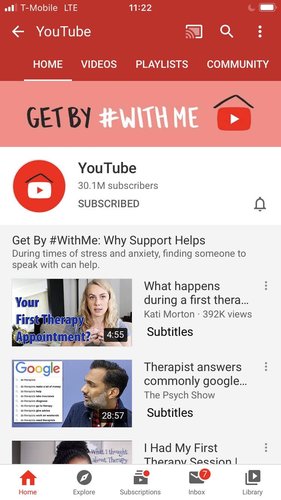A person is using their phone, as indicated by the T-Mobile network status, signal strength, and icons along the top of the screen. The time displayed is 11:22 and the battery bar shows a mostly full charge.

The screen shows the YouTube app open on the home tab, indicated by a white arrow pointing left, labeled "YouTube," and a highlighted "Home" option with a line underneath it. Other visible tabs include "Videos," "Playlists," and "Community."

A red and black banner at the bottom reads "Get By #WithMe," referring to a YouTube hashtag campaign with 30.1 million subscribers. 

Below this, there is a gray box with text promoting support during stress and anxiety, mentioning the importance of finding someone to talk to: "Why support helps during times of stress and anxieties. Finding someone to speak with can help."

Following this, there is a featured video by Kati Morton titled "What happens during a first…," presumably about therapy, with 392,000 views and subtitles. The video thumbnail shows Kati Morton, a blonde-haired woman, speaking, and is 4 minutes and 55 seconds long. The blue text next to the thumbnail reads, "Your first therapy appointment."

Immediately below this is another video titled "Therapist answers commonly googled…" from "The Psych Show" with subtitles. Lastly, the bottom-most video is titled "I had my first therapy session."